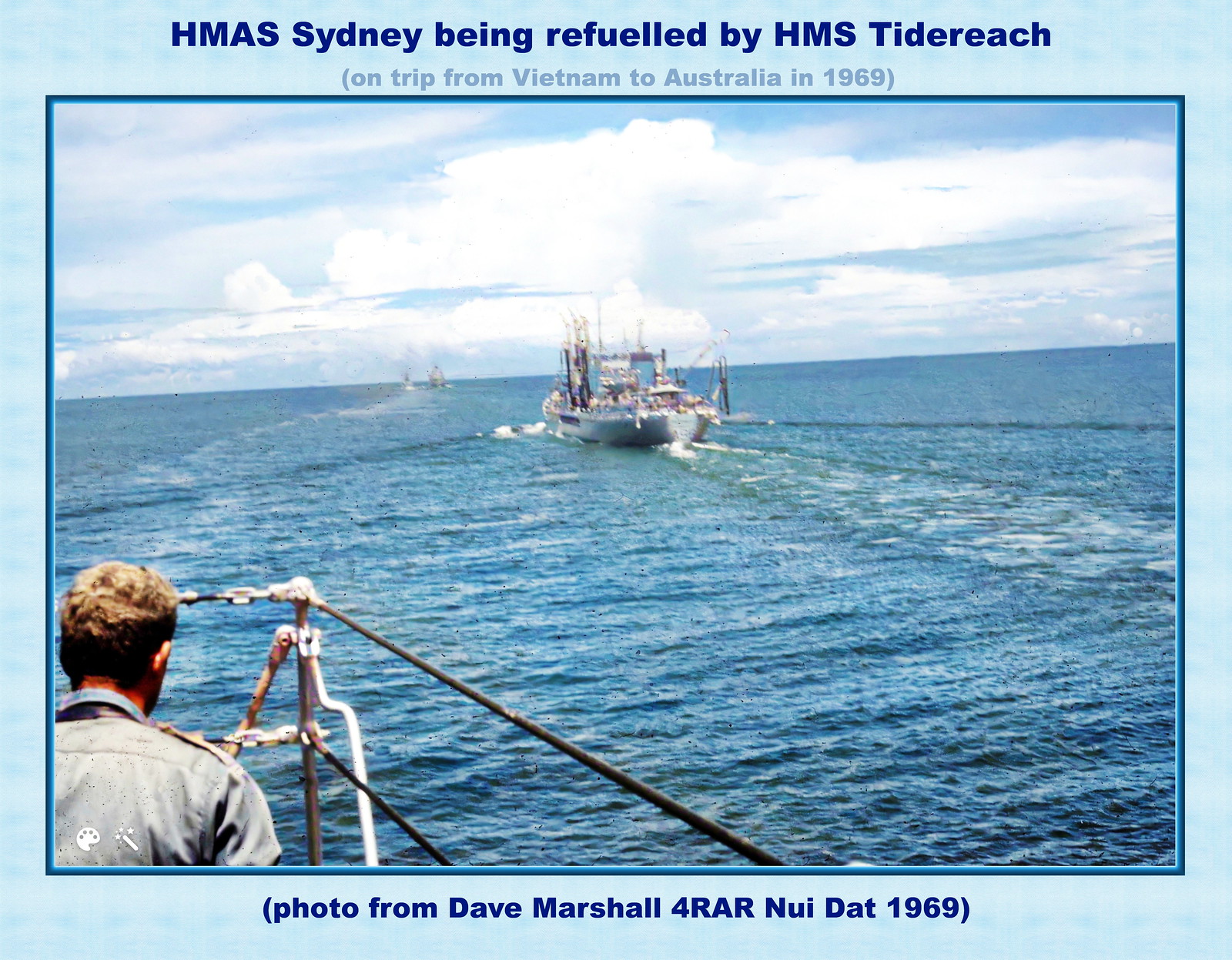The photo titled "HMAS Sydney being refueled by HMAS Tyridge on trip from Vietnam to Australia in 1969" shows a detailed scene on the open ocean. The image features a large white ship, positioned centrally, identified as being refueled mid-voyage. The ship's two prominent structures extend skyward from its deck, and it's in motion, as evidenced by the white waves trailing behind it. The expansive sky, occupying the top third of the image, is a vibrant blue adorned with scattered white clouds.

In the foreground, visible in the lower left corner, stands a man dressed in a gray uniform with short brown hair. He is positioned behind a wire fence on what appears to be another vessel, facing towards the refueling ship. His posture and gaze suggest he is observing the operation. Surrounding the image is a light blue border, with text indicating the title and details of the event, including the notation "Photo from Dave Marshall, 4 RAR, Noy Dat, 1969." The overall scene is set under clear daylight, capturing a significant naval moment during the Vietnam War era.